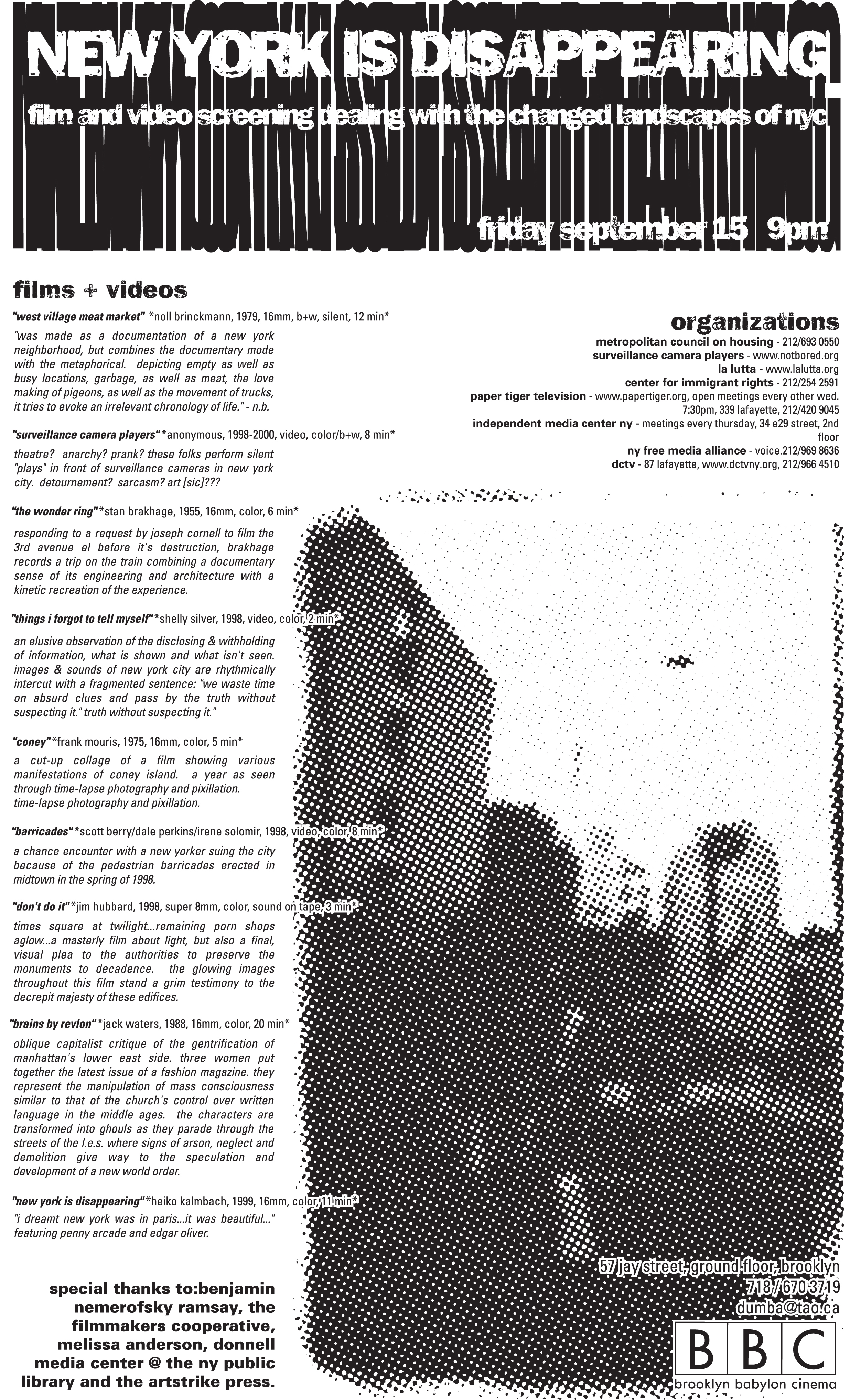This detailed black-and-white poster, intentionally designed with a vintage look, announces a film and video screening titled "New York is Disappearing." It explores the transformed landscapes of New York City and is scheduled for Friday, September 15th, at 9 PM. The poster resembles a newspaper or magazine page, laden with small, densely-packed text that includes a blurry, pointillist-style image of a decayed and abandoned New York City landscape, reflecting the event's theme. A black header at the top bears the event title in white text. Below the header, the poster lists filmmakers, years, and formats of the featured works on the left side, while the right side houses a section dedicated to various participating organizations, including their contact information. At the bottom right, the text "BBC" stands for Brooklyn Babylon Cinema. Additional recognition is given to several contributors: Benjamin Nemirovsky Ramsey, the Filmmakers Cooperative, Melissa Anderson, Donnell Media Center at the NY Public Library, and ArtStrike Press.